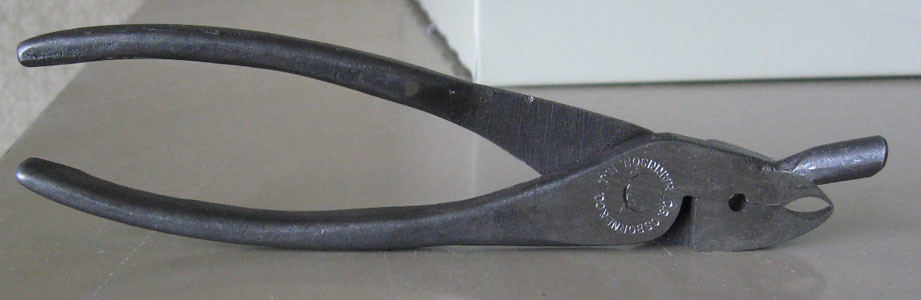This is a highly detailed photograph of a metal tool that appears to be a pair of pliers, positioned upright on its side and facing right. The tool is made of grayish-silver, shiny metal and features two handles that start on the left side of the image, gradually spreading apart before coming together. These handles converge towards the head of the tool, which is equipped with a sharp, pointed end and a small welded silver piece. Near this welded part, there's an engraving in a circular, clockwise pattern, although the text within this embossing is indistinguishable due to the lighting. The pliers are closed and rest on a gray table or counter, set against a white background which is likely a wall. Additionally, a cylindrical silver extension, roughly an inch long, protrudes from the top of the pliers, adding to the complexity of the tool's design.